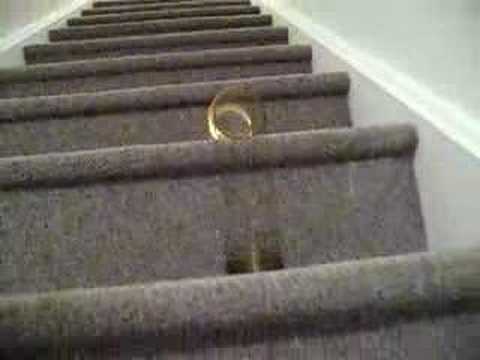This photograph captures a staircase, carpeted in gray, extending upward with walls on both sides that are either white or light blue. The image appears somewhat grainy or pixelated, resembling a still from a video. The second step from the bottom features a knocked-over glass, positioned with its opening facing towards the viewer. Visible streaks of liquid run down from the glass, creating darker stains on the carpet, especially where the liquid has pooled at the base of the stairs. Additionally, there is a gold or silver slinky descending the staircase, captured mid-movement, although the focal spill and its resultant stain draw the most immediate attention. The lip of each step is subtly defined, and the side walls are complemented by white baseboards running parallel to the staircase. Thus, the photograph intricately documents both the accident involving the glass and the playful presence of the slinky amidst the domestic setting.